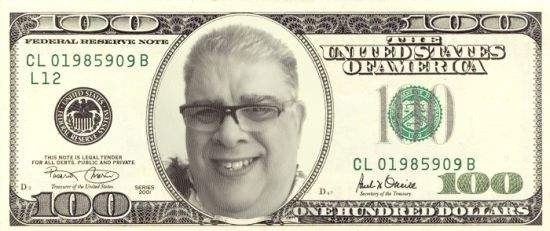This photograph features a $100 bill that has been altered to replace Benjamin Franklin with a new figure—a large man with light-colored spiky short hair, approximately an inch long, wearing sunglasses. The man has a big smile, displaying nice teeth. His sunglasses have black frames at the top but no frames at the bottom, giving them a half-rim appearance. The design of the bill retains its original elements, including "The United States of America" at the top, the green Treasury seal, the number "100" at the bottom, and the serial number CL 01985909BL12. The alteration seems to be a playful edit, possibly done as a joke or hobby, and the man's face is oriented towards the left side of the image. The bill also bears the signatures of the Treasury and detailed yet unreadable fine print. The overall look maintains the $100 bill’s traditional black, cream, and green color scheme.